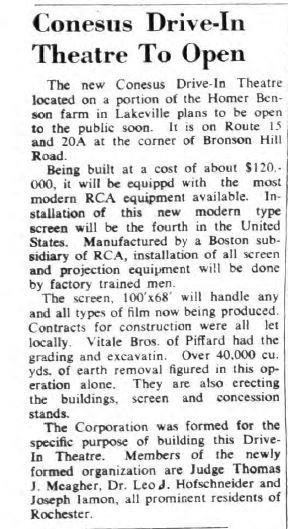This image is a photograph or scan of an old article. The article's background is white with black text. The title, in large bolded black text, reads "Consensus Drive-In Theater to Open." Below the title are several paragraphs in smaller text detailing the grand opening of the new Consensus Drive-In Theater, which is situated on a portion of the Homer Benson Farm in Lakeville, at the intersection of Route 15 and 20A and Bronson Hill Road.

The article highlights that the drive-in theater is being constructed at an estimated cost of $120,000 and will feature state-of-the-art RCA equipment. Notably, this will be the fourth installation of the new modern type screen in the United States, manufactured by an RCA subsidiary in Boston and installed by factory-trained technicians. The screen, which measures 100 inches by 68 inches, is designed to handle any film currently in production.

Local contractors have been employed for the construction work. The Tally Brothers of Pifford are responsible for the grading and excavating, a significant task that involved removing over 40,000 cubic yards of earth. They are also erecting the building, screen, and concession stands. 

The article mentions that a corporation was formed specifically to build this drive-in theater, with its members including Judge Thomas J. McAher, Dr. Leo J. Hofschneider, and Joseph Lemon, all of whom are prominent residents of Rochester.